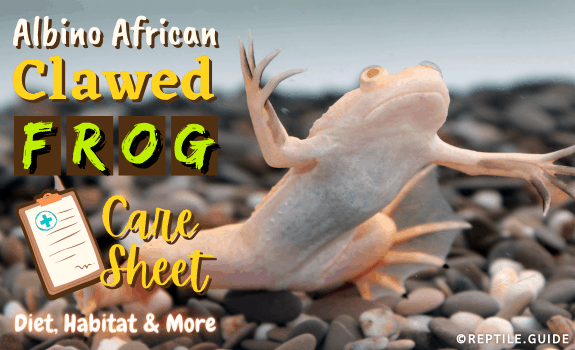The underwater scene depicts an albino African clawed frog, characterized by a predominantly white body with subtle peach and beige hues, including soft orange accents on its upper limbs. The frog appears to be energetically propelling itself upwards from a gravel surface, which consists of a mix of gray and white pebbles. Its large webbed feet are evident, aiding in its swimming motion. The background, although blurry and muted in shades of blue and grey, helps highlight the sharp focus on the frog and the foreground details. The top left corner features text in various colors, organized as follows: "Albino American Clawed Frog" in white, "Care Sheet" in yellow, with a clipboard icon and a blue Red Cross-style sign, and "Diet, Habitat, and More" in white. The copyright "reptile.guide" is conspicuously placed in the lower right-hand corner, framing this educational and visually striking photograph.